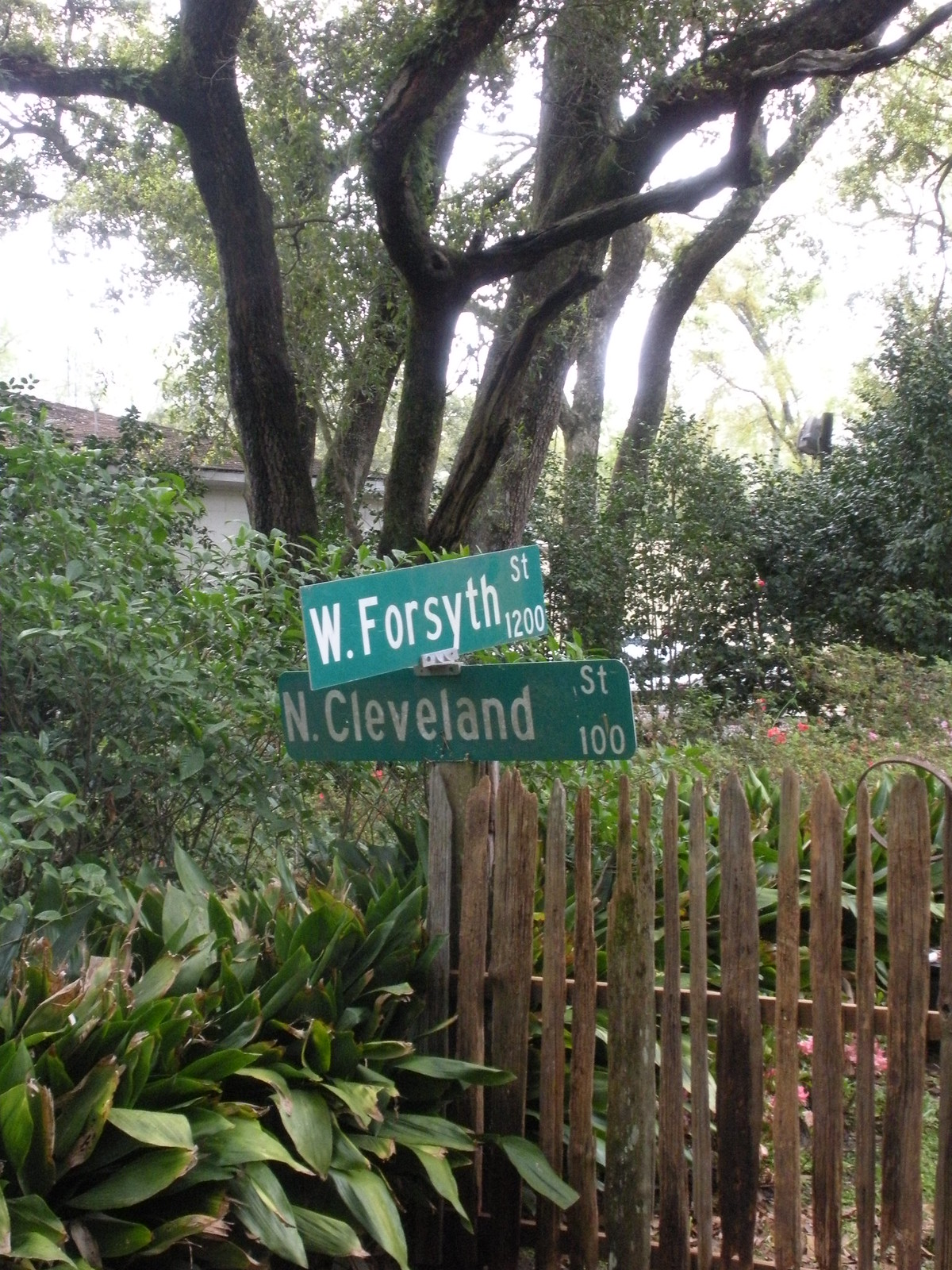In this picturesque backyard garden, a large brown tree and several smaller ones dominate the upper portion of the image, their branches elegantly arching overhead. A lush assembly of green shrubs and plants flanks both the top right and left sides of the scene, creating a verdant frame. Adjacent to the cluster of greenery on the left is a section of a roof and a pristine white wall. The lower left corner features smaller, vibrant green plants, adding to the botanical diversity. A distinct street sign, positioned either atop or beside a light brown fence on the right, directs viewers to West Forsyth Street 1200 and North Cleveland Street 100. The signs themselves are a contrasting green with clear white lettering. The overall scene captures a harmonious blend of natural elements and urban markers, framed by the comforting embrace of the garden's flora.